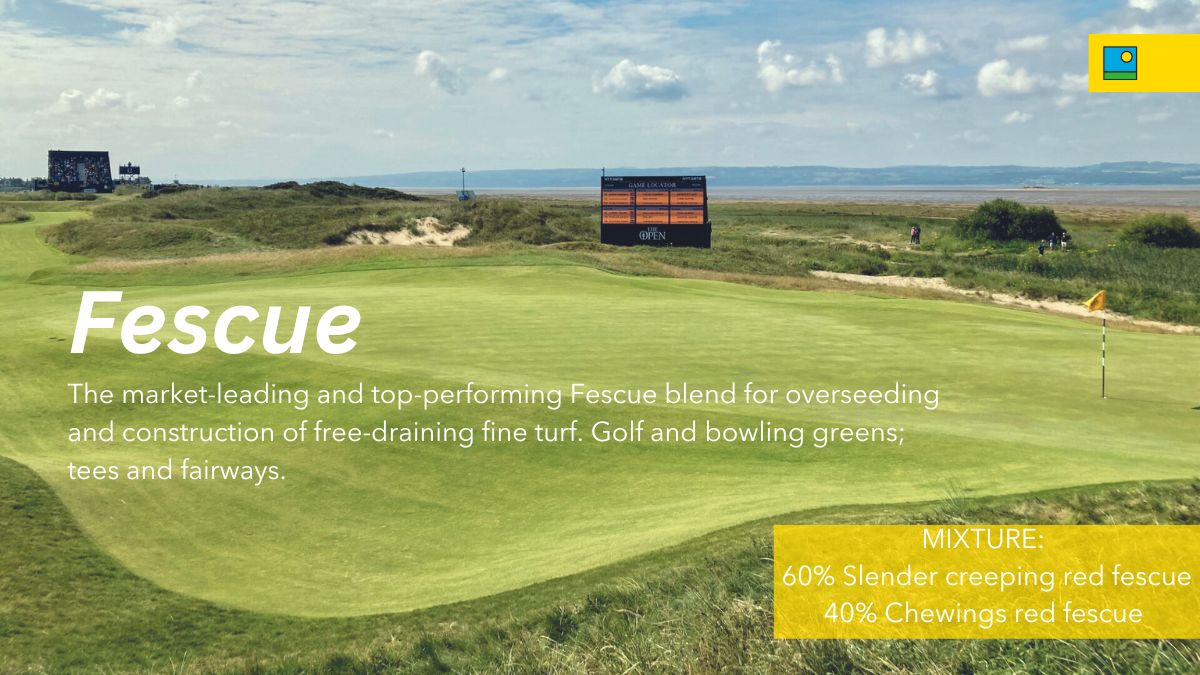The image depicts an advertisement for Fescue blends, set against a scenic golf course backdrop. The field is lush and green, bordered by grasses and shrubs, and it's a bright day with puffy white clouds scattered across the blue sky. In the top right corner, there is a yellow bar and a blue disc with a hole revealing an orange section, while the bottom features a green bar. Central to the image is a black and rust-colored structure. Overlaid on the scene is prominent text reading "Fescue," highlighting it as the market-leading and top-performing blend for overseeding and constructing free-draining fine turf, suitable for golf and bowling greens, tees, and fairways. Additional smaller text specifies the mixture as 60% slender creeping red fescue and 40% chewing red fescue.